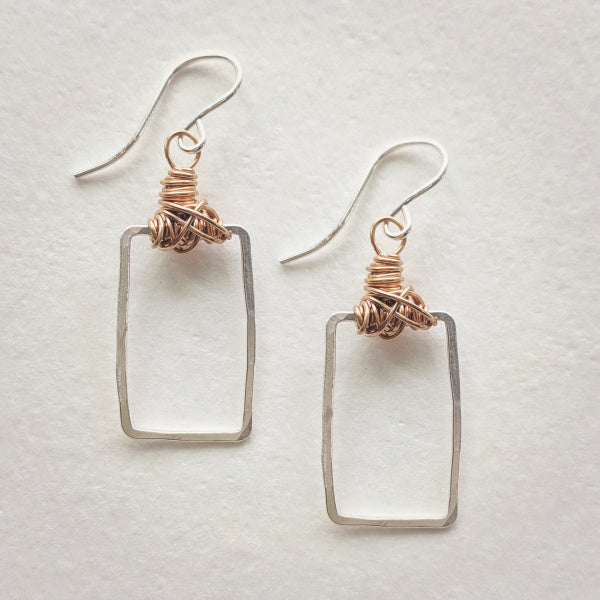This image displays a pair of handmade earrings set against a white textured background, possibly paper. The earrings are crafted using two types of metal, giving them a distinct two-toned appearance. Each earring features a vertical, open rectangular frame made of hammered silver, showcasing slight irregularities typical of handcrafted items. At the top of each rectangle is an intricate cluster of tightly coiled copper wire, wrapped multiple times around itself, forming an ornamental and eye-catching design. The earrings are suspended from traditional shepherd's hooks ear wires made of the same silver-toned metal as the rectangles. The image shows the earrings lying on the white surface, with the one on the right positioned slightly lower than the one on the left.